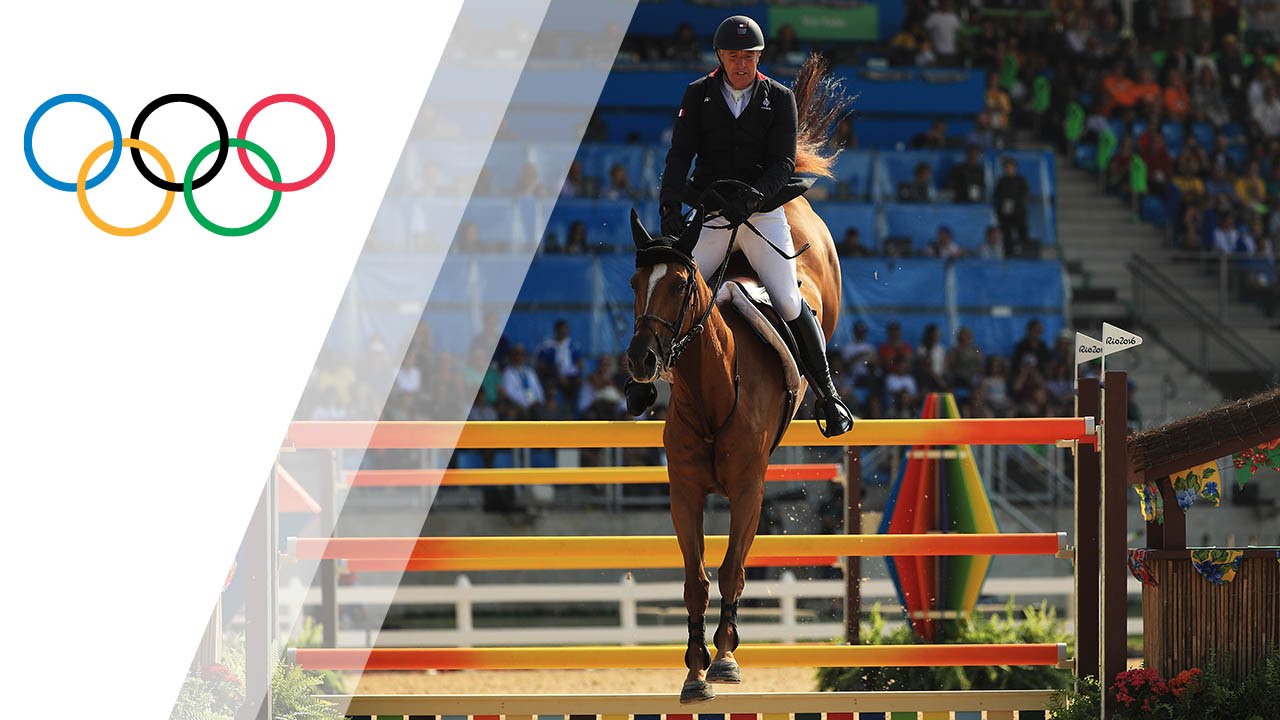This is a detailed color photograph capturing a dramatic moment in an Olympic equestrian event. The rectangular image showcases a brown horse with a white blaze leaping over a red and yellow fence. The horse, adorned with black reins and a white saddle blanket, is being skillfully ridden by a man standing on the stirrups, clad in knee-high black boots, tight white pants, a black riding jacket, and a round cloth-covered jockey's helmet. His focused expression reflects the intensity of the steeplechase event. In the top left corner, the iconic five interlocking rings of the Olympic symbol—blue, yellow, black, green, and red—are prominently displayed against a white triangular banner. The background reveals a grandstand filled with spectators seated in blue chairs, intently watching the thrilling action unfold.